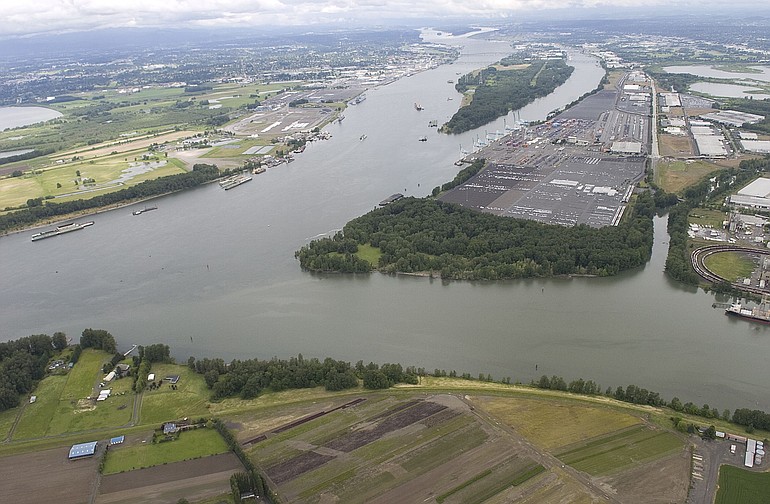An aerial panoramic photograph captures a sprawling landscape that appears to be taken from a high vantage point, possibly from a plane, helicopter, or drone. The central focus of the image is a large, dark greenish-gray river with several barges navigating its waters, surrounded by extensive industrial landmasses interspersed with patches of trees. On the right side of the image, dense woods and shrubbery are visible, while a network of roadways and parking lots, characterized by extensive blacktop surfaces, sprawls across the scene. Farmlands and numerous tiny buildings are also noticeable in the bottom portion of the image. Toward the back of the photograph, a cityscape rises against a gloomy, overcast sky painted in shades of blue and white, enhancing the industrial ambiance. Additionally, the visual includes open expanses of concrete, warehouses, some train tracks, and hints of a possible airport base or campus-like structure. The overall setting conveys a non-residential, utilitarian environment with considerable space between structures.